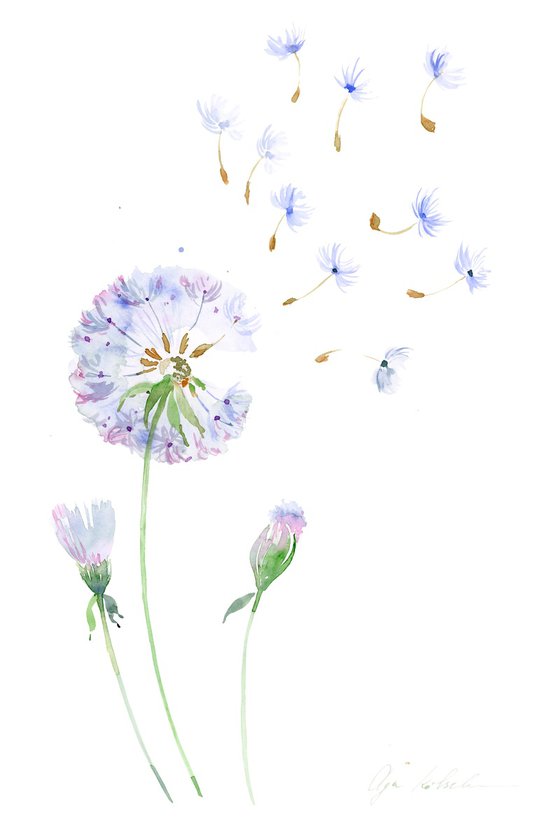The image is a whimsical digital drawing depicting a trio of wildflowers against a completely white background. On the bottom right, faintly sketched in cursive with light purple ink, is the artist's initial, although it is too blurry to decipher. The focus of the artwork is on the left side, where three flowers with green stems are illustrated. The central flower has fully blossomed, forming a circular shape with purple-pink petals. Flanking this central bloom, the two adjacent flowers remain in their budding stages, yet to open. Adding to the delicate and airy feel of the piece, small blue and brown dandelion spores float above the flowers, evoking a sense of gentle dispersal and whimsy.